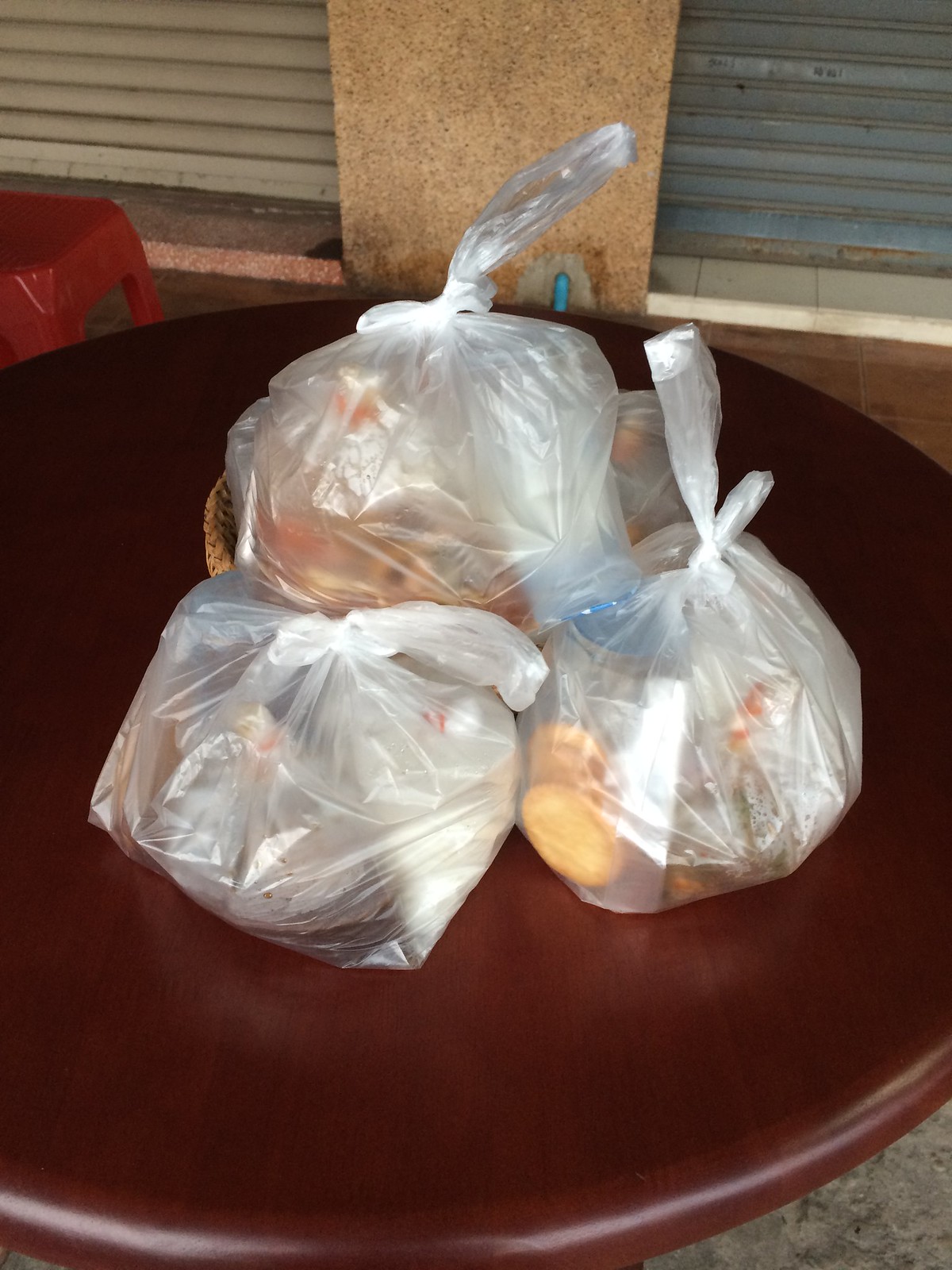The image features a round, dark brown wooden table with three semi-opaque plastic bags tied at the top, arranged in a small pyramid with one bag stacked atop the other two. The contents of the bags are unclear, but there are hints of different colors and objects: the bottom right bag contains light-colored, cookie-shaped objects with some reds, greens, and blues visible, while the left bag has white and dark colors with a touch of red. The top bag, possibly sitting in a golden-colored basket, also shows red and white. In the background, a red plastic chair is located in the upper left corner, and a stone-flecked cement rectangular post is in the center. Flanking the post are two silver roll-up doors, commonly used to secure restaurant or store entrances. The room floor appears to be of gray marble, and contrasting materials suggest different windowsills on each side of the post, one of light tile and the other of red marble.